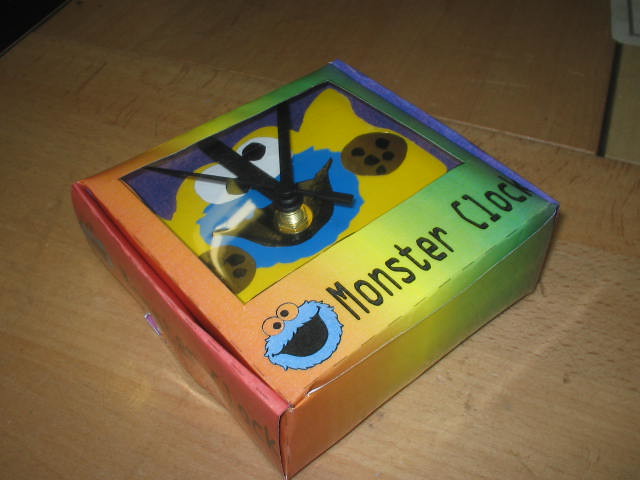The image showcases a vibrant, nostalgic Cookie Monster clock placed on a wooden desk. Encased within a square, multicolored box, the design features a striking rainbow gradient transitioning from red to orange, yellow, green, blue, and finally purple as one moves from left to right. Prominently displayed at the bottom of the box in bold black letters is the inscription "Monster Clock." The clock face captures Cookie Monster with his iconic googly eyes positioned at the 12 o'clock mark. Flanking Cookie Monster are two tempting chocolate chip cookies, one on each side. The background behind him is reminiscent of a Rorschach test, with a yellow splotch layered over a purple one, adding a playful, abstract touch. The black clock hands indicate the time as precisely 12 o'clock.